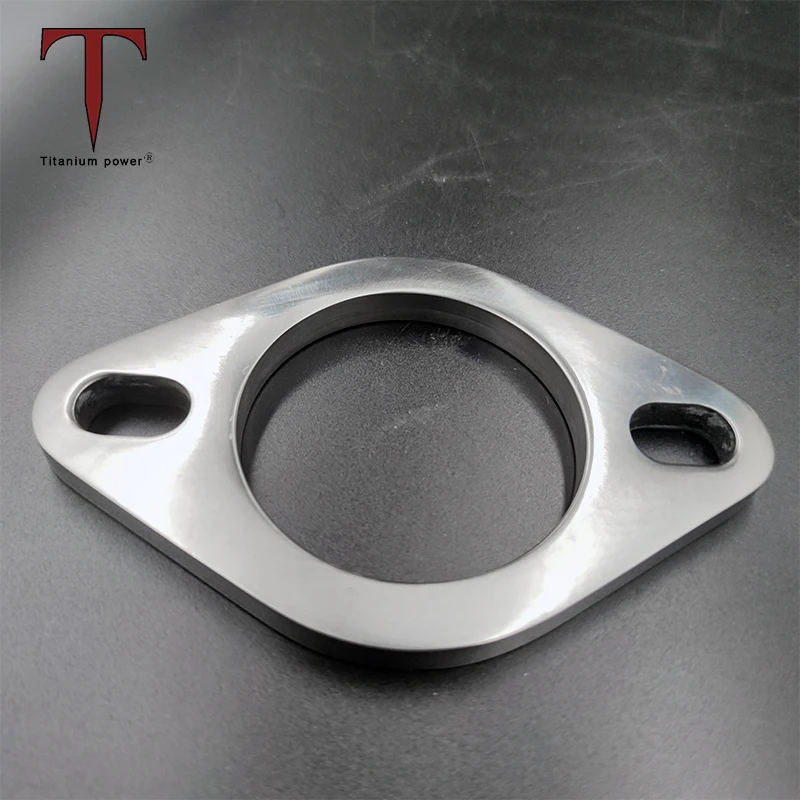This is a detailed close-up photograph of a metal object positioned on a dark gray, slightly scratched surface. Dominating the upper left-hand corner is a prominent red T with a pointed bottom, accompanied by the words "Titanium Power" and a registered trademark symbol. The metal object itself is thick, silver-toned, and resembles a curved diamond or a peach shape. Centrally, it features a large circular cutout, flanked by two elongated oval openings at each end, suggesting the item might be a specialized car part or a component with aerodynamic applications. The image, taken from a top-down perspective, emphasizes the object's robust, metallic construction against the stark, contrasting background.